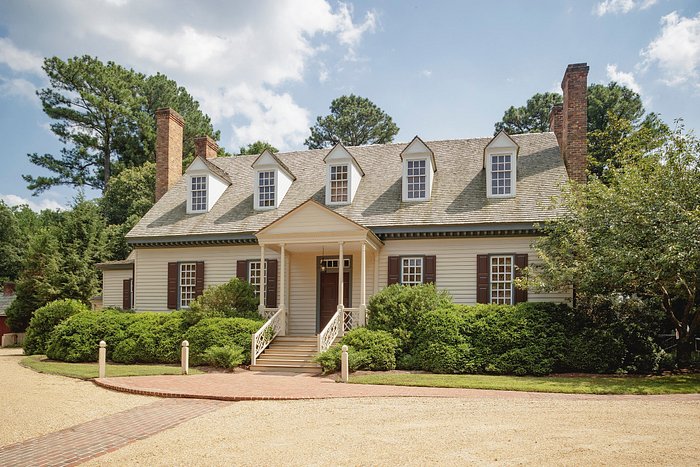This image features a Victorian-style, single-story house located in a suburban neighborhood. The house is painted a light color, possibly white or beige, and has a distinctive gray roof adorned with five evenly spaced dormers. Each dormer has a window that is likely intended for light and aesthetic purposes rather than as living spaces. Flanking the roof are four tall brick chimneys, two on each side, which add to the house's old-world charm.

The symmetrical façade has four large windows with box-patterned panes, two on either side of the centrally located front door. The entryway is covered by a small porch with its own roof and leads to a set of steps that descend to a brick walkway and driveway. This front area is landscaped with neatly trimmed shrubs, and the yard includes a well-maintained patch of grass bordered by a row of hedges. 

In the background, there are three trees—one on each side of the house and one behind it in the center—that frame the property and add a touch of natural beauty to the scene. The house sits adjacent to a brick and gravel road or driveway, which appears to be a quiet, activity-free suburban street.